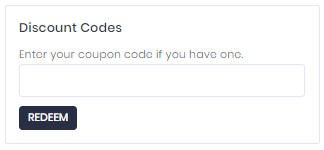The image depicts a minimalist coupon code entry box designed in a compact, rectangle shape resembling the dimensions of a credit card but narrower. The box features a subtly faded gray border outlining its shape against a clean backdrop. Positioned in the upper left-hand corner, the text "Discount Codes" appears prominently in bold black font. Below this, an instructional phrase is displayed in a lighter grayscale: "Enter your coupon code if you have one."

Dominating the center of the image is a wide, blank, white input field, intended for users to type in their coupon codes. At the bottom left-hand corner of the box, there is a clickable black button labeled "Redeem" in bold, capitalized white letters, designed to confirm the coupon code entry. The remainder of the box, spanning from the center to the right-hand side at the bottom, is filled with blank white space, emphasizing the simplicity and focus of the form's purpose. The overall design is geared towards functionality and ease of use.